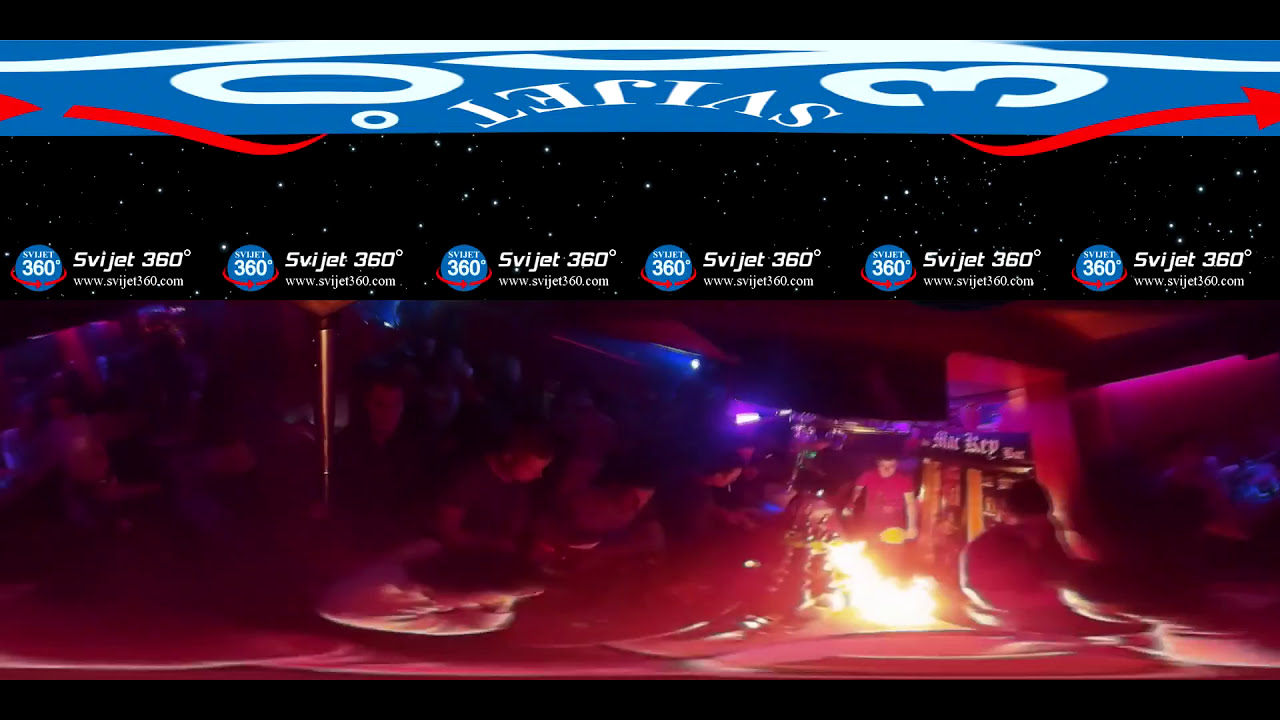The image is a 6-inch wide by 3-inch high, highly distorted and warped photo, likely captured by a 360-degree camera. The scene appears to be taken indoors, possibly in a local food eatery or bar, with a darkened atmosphere. On the bottom, a crowd of people can be seen gathered around what looks like an open flame on a long grill, suggesting a cooking area. Coolers and other bar-related elements are visible in the background. 

At the top of the image, there are multiple banner layers providing logos and text. The topmost layer features a narrow black band, followed by a blue band with a white stripe. This layer includes white upside-down text "SVIJET 360" and other letters. Below it, a black banner with white stars aims to emulate the sky or universe. 

A repeated logo appears six times across the banner, consisting of a blue circle with a red arrow circling around it, alongside the text "SVIJET 360 degrees" and the URL "www.svijet360.com". This logo is also present on the top right, with similar details. The overall low-quality and distorted nature of the image gives it a super skewed, rounded appearance. At the bottom left, partially legible signage suggests a place name, potentially "MAC KEY bar".